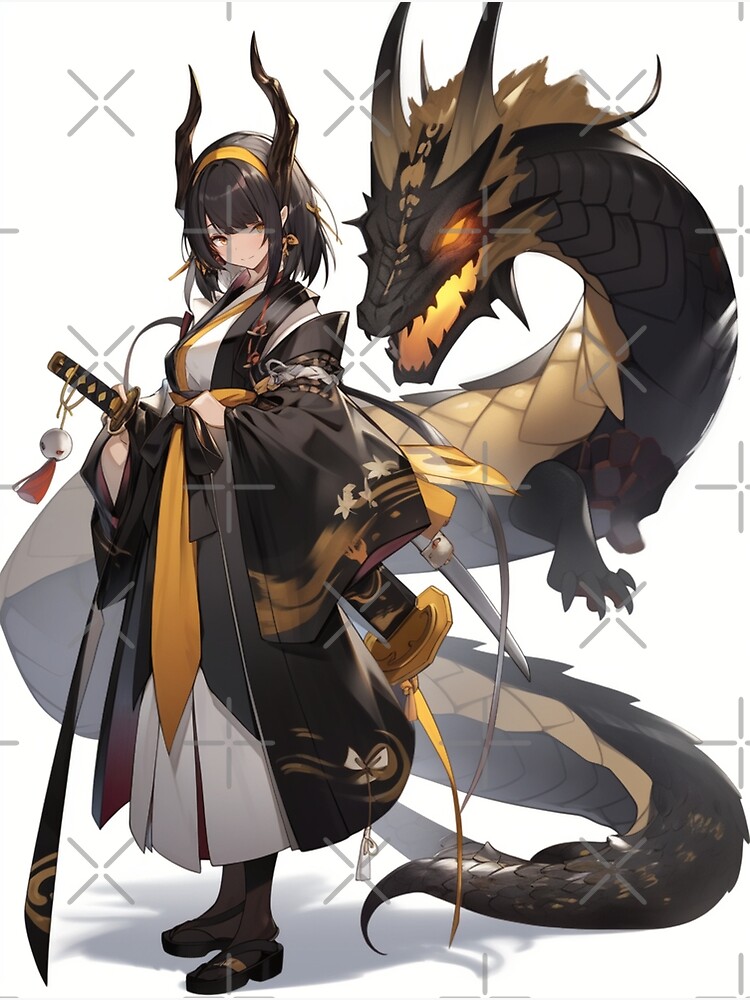This vibrant anime illustration features a poised warrior girl and a majestic dragon set against a white background. The girl, adorned in a black, gray, and gold kimono with a yellow scarf and black kimono shoes, carries a sheathed katana and another sword with a white circular charm. Her shoulder-length black hair is complemented by a yellow headband and black antler-like horns, giving her a seductive yet formidable appearance. Standing slightly ahead, she has a blushing, determined face that hints at her role as a heroine or warrior. Behind her, the imposing black dragon with glowing orange eyes and a fiery mouth adds an intense aura. Its lithe, flowing body, covered in yellow-scaled underbelly and crowned with light brown horns and mane, coils protectively around the girl. Star-like crisscross patterns overlay the image, adding a watermark effect, enhancing its dynamic and mystical feel.